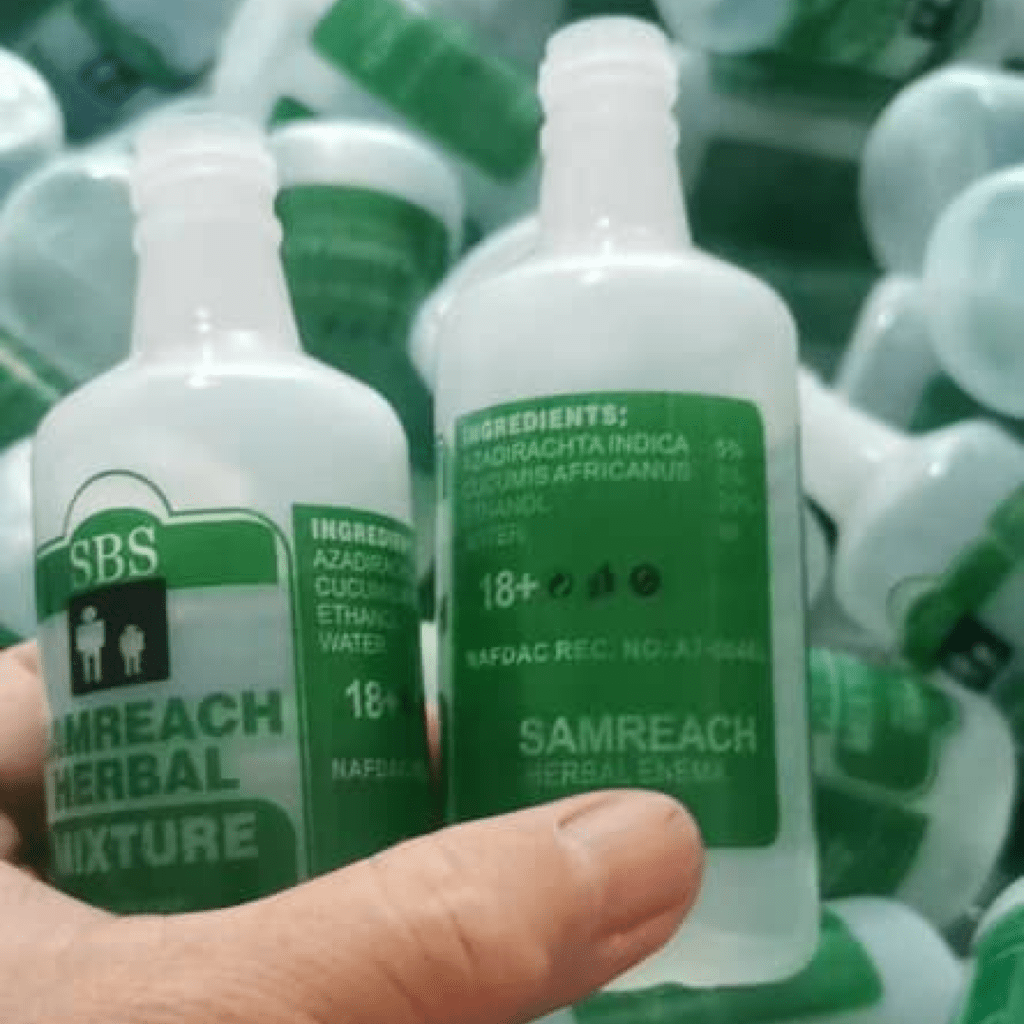This indoor photographic image captures a close-up of a person's white hand holding two cylindrical, clear plastic bottles of the same size and shape. Both bottles feature green labeling with curved edges but lack caps. The left bottle's front label displays an intricate design: a semi-circle at the top with the text "SPS M Reach Herbal Mixture." Below this, a black square contains hazy illustrations, possibly of a larger and smaller person, and fragmented text that partially reads "AZAD..." and "CUCIR..." along with "ethanol water 18 plus." The right bottle sports an all-green rectangle, flaunting the full ingredients list, though it's too blurred to discern. Notably, it highlights "18 plus," "Samreach Herbal," and the brand name "Samreach." Surrounding these centered bottles, the out-of-focus background showcases a multitude of identical bottles stacked in a densely packed arrangement.